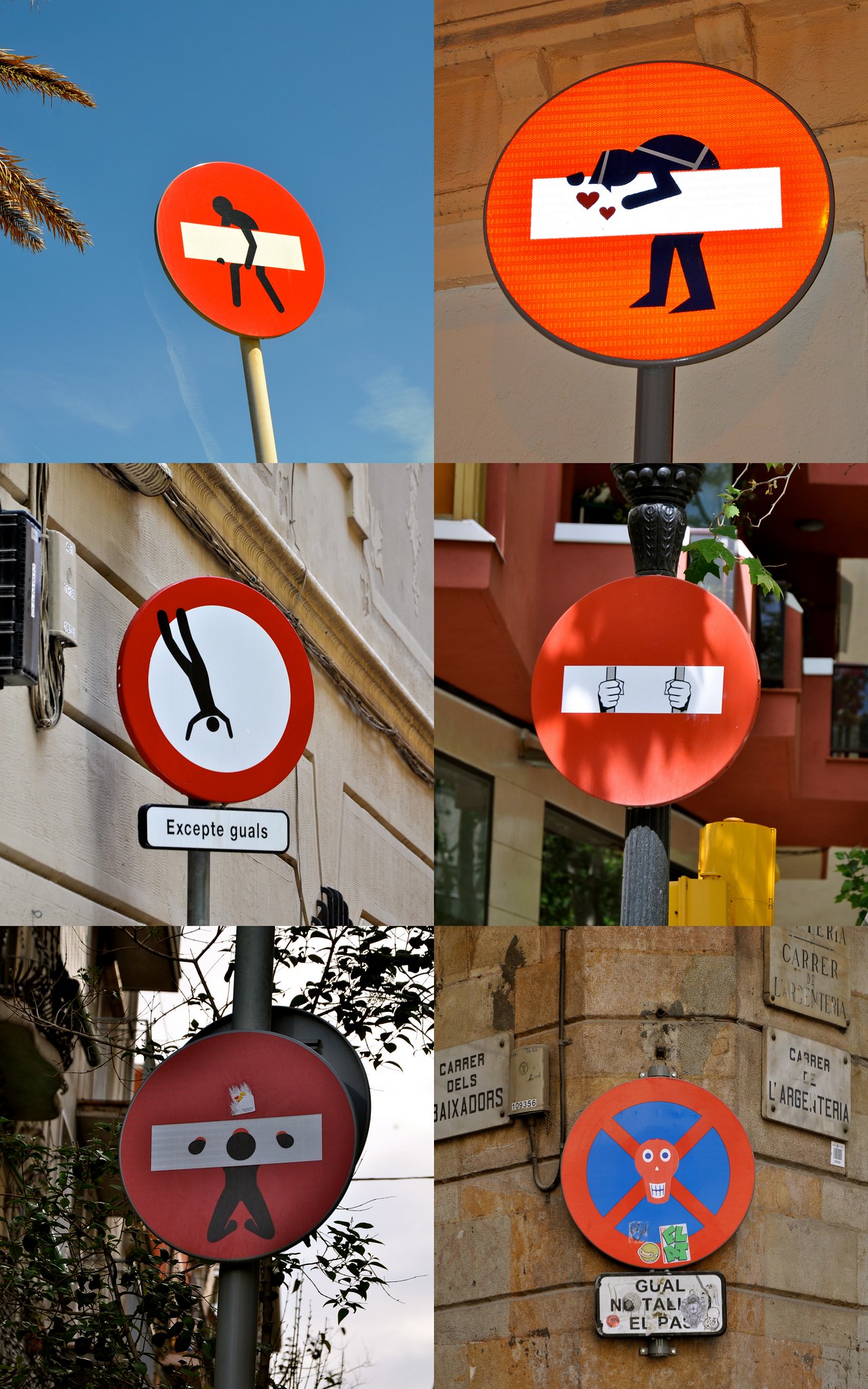The image is a vertical rectangular compilation of six humorous photos featuring creatively altered road signs, arranged in two columns of three. Each photograph displays a red sign with whimsical artwork applied, resembling yield or no entry signs. The signs are adorned with black illustrations of people interacting with the white bars typically found on such signs.

- Top left: A person appears to be carrying the white bar of the sign.
- Top right: A man with a cap is seen kissing the white bar, which contains three small red hearts.
- Middle left: Two hands grip the white bar, resembling prison bars.
- Middle right: A figure somersaults, creating the illusion of falling into a hole.
- Bottom left: A figure behind a white bar, resembling a stockade.
- Bottom right: A no entry sign with a red skull motif.

These amusing modifications transform ordinary signs into lighthearted visual gags. The signs are located on city streets with high-rises, and the surrounding text suggests a Spanish-speaking country, with a building marked "Carrere de Baxadores."